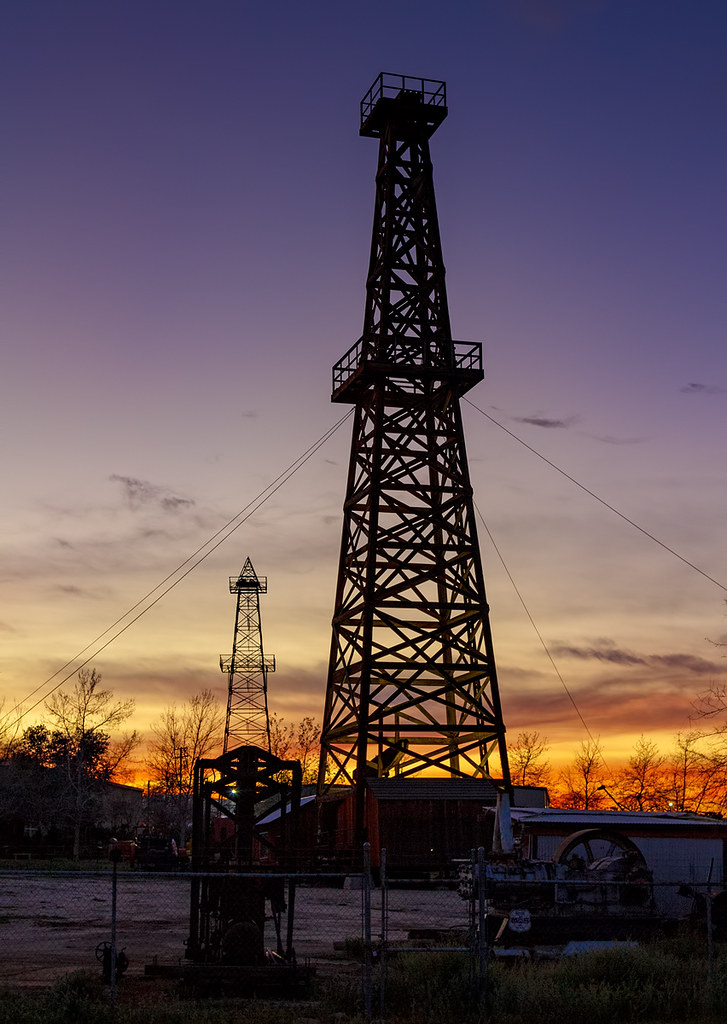In this photograph, taken during a vivid sunset, there is a tall oil rig tower featuring multiple cross beams and stabilizing wires, four in total, two on each side, ensuring its stability. The sky transitions from bright orange hues near the horizon to darker blue and purple tones with a few wispy clouds scattered about. Surrounding the tower, which resembles a cell phone tower, are various pieces of oil well machinery, including a large wheel with spokes and a fenced perimeter. There are also buildings visible; a small white structure on the right and a reddish structure at the tower's base that almost looks barn-like. In the foreground, there's some grass, partially obscured by the encroaching darkness, and potentially a truck or a shed. In the background, another similar tower stands silhouetted against the sky. Between the top and bottom sections of the primary tower, a maintenance basket is visible, possibly used by workers. The overall scene is bathed in the rich, warm light of the setting sun, blending into the deepening twilight above.